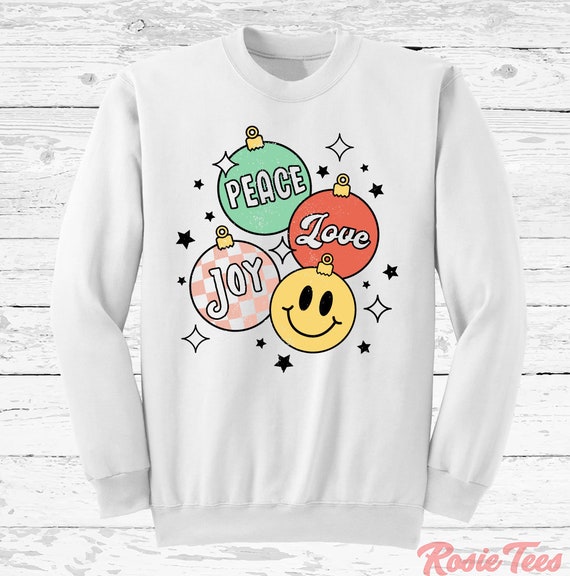This image showcases a white sweatshirt displayed against a rustic, painted white wood background. The sweatshirt features four Christmas ornaments, each with a distinct design and message. The ornaments include a green one labeled "peace," a reddish-orange one labeled "love," a pink and white checkered one labeled "joy," and a yellow smiley face with black eyes and a smile. Surrounding the ornaments are small black stars and square shapes resembling sparkles. In the bottom right corner, the sweatshirt is marked with "Rosie Tease" in pink, cursive-like lettering. The overall design appears tailored for a festive, perhaps slightly feminine audience, though it offers versatile appeal.